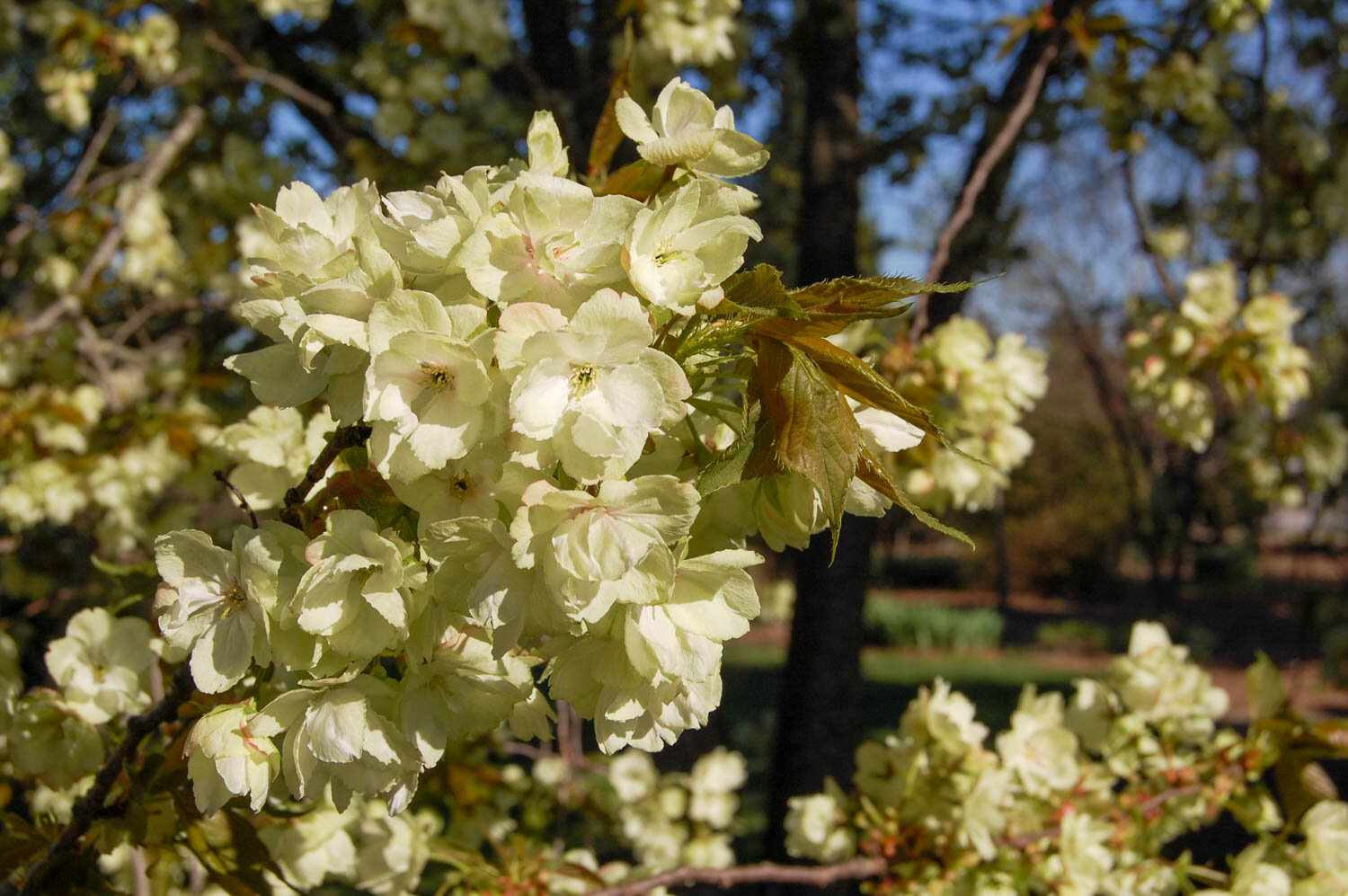This image captures a close-up of a flowering tree branch, showcasing the delicate, predominantly white flowers tinged with light yellow and a subtle hint of pink in their centers. The clusters of flowers enhance the tips of the branches, while the reddish-brown to olive green leaves form a contrasting backdrop. The tree, appearing to have just bloomed in the early spring, stretches out with multiple branches, some in sharp focus and others softly blurred in the background. The clear blue sky without any clouds adds a serene ambiance to the scene, highlighting the vibrant, fresh appearance of the flowering tree.